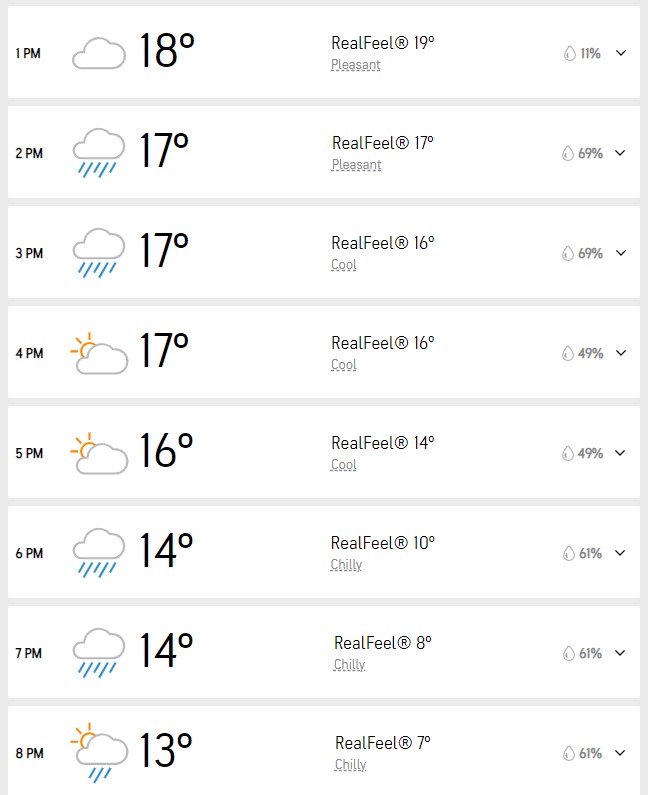Here's a detailed and cleaned-up caption based on the voice description provided:

---

**Weather Forecast**

- **1:00 PM**: Cloudy skies with a temperature of 18°C; it feels like 19°C. There is a 11% chance of rain.
- **2:00 PM**: Rain clouds appear with a temperature of 17°C, matching the real feel. Pleasant weather with a 69% chance of rain.
- **3:00 PM**: Continued rain with a temperature of 17°C; it feels like 16°C. Cool weather and a 69% chance of rain.
- **4:00 PM**: Partly sunny with intermittent clouds at 17°C, feeling like 16°C. Cool conditions and a 49% chance of rain.
- **5:00 PM**: Partly sunny with a temperature drop to 16°C; it feels cooler at 14°C. Slightly brisk with a 49% chance of rain.
- **6:00 PM**: Rain resumes with a temperature of 14°C, and it feels like a chilly 10°C. There is a 61% chance of rain.
- **7:00 PM**: Rain continues, maintaining 14°C but feeling much colder at 8°C. Chilly conditions persist with a 61% chance of rain.
- **8:00 PM**: Light rain with partial sunshine, temperature at 13°C, feeling like a very chilly 7°C, and a 61% chance of rain.

---

This detailed weather forecast provides an hour-by-hour breakdown of the temperature, real feel, and chance of rain, helping to prepare for the day's varying conditions.